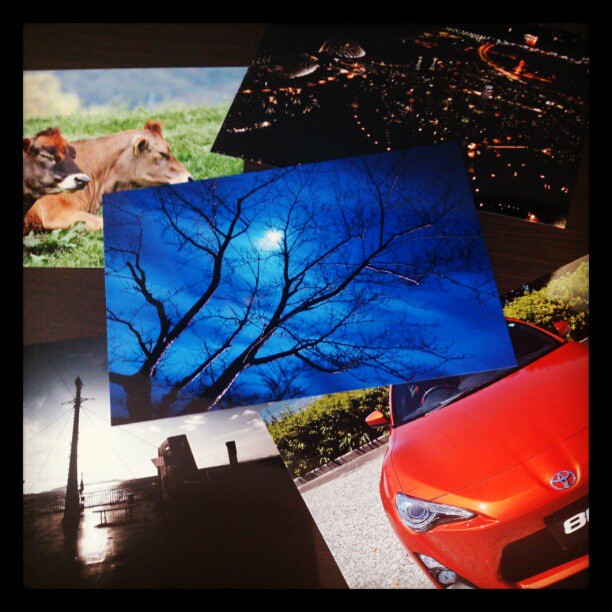The image is a detailed collage of five distinct photographs artfully laid out on top of each other. At the center top is a striking image of a blue night sky illuminated by the moon, casting its glow onto a solitary, leafless tree with branches stretching outward. Directly below this, a vibrant red Toyota car with a sporty design is captured up close, featuring a center oval emblem, a black grill, a number 8 license plate, and triangular headlights. The car rests on a gravel or dirt surface with a hedge wall behind it. To the left of the tree image is a shadowy landscape, and at the upper left corner, two cows—one black and one light brown—are shown lying on green grass under a cloudy sky. The top right corner presents a captivating aerial view of a city at night, its buildings aglow with lights against the dark sky. The bottom left of the collage appears to feature an early morning scene of a pier with a telephone pole silhouetted against the sky, which isn't explicitly detailed but inferred from the descriptions.